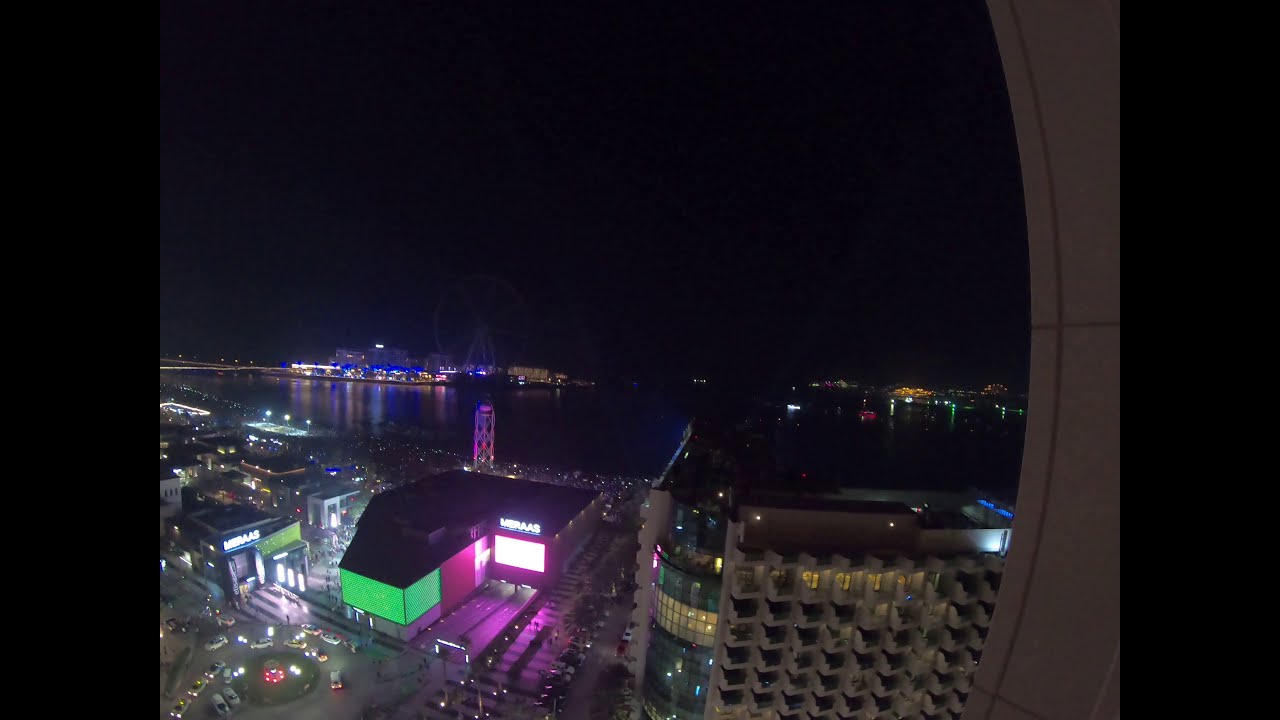This detailed night-time aerial photograph of a vibrant cityscape, possibly taken from a plane window, captures a bustling urban area illuminated by neon lights and streetlamps. The image is horizontally rectangular with vertical black stripes on both sides, suggesting the perspective is framed by a window. 

Central to the image is a dark body of water, likely a river, reflecting the surrounding lights. A bridge can be faintly discerned stretching over the water. In the distance, a ferris wheel adds an element of whimsy against the dark sky, accompanied by various illuminated buildings. 

The bottom section reveals a complex road network crowded with cars and bright traffic lights. On the right side, a 10 to 12-story building with balconies, possibly an apartment complex, stands prominently. Adjacent to this building is a street leading to another structure with distinctive architecture: it features vivid lime green and magenta neon sides and a bright white sign on its roof. 

Additional buildings, varying in height with the tallest resembling a hotel, showcase multicolored lights on their facades, contributing to the scene's lively atmosphere. The chaotic mix of glowing signage, heavy traffic near a roundabout, and residential and commercial structures creates a vivid and dynamic snapshot of city life at night.